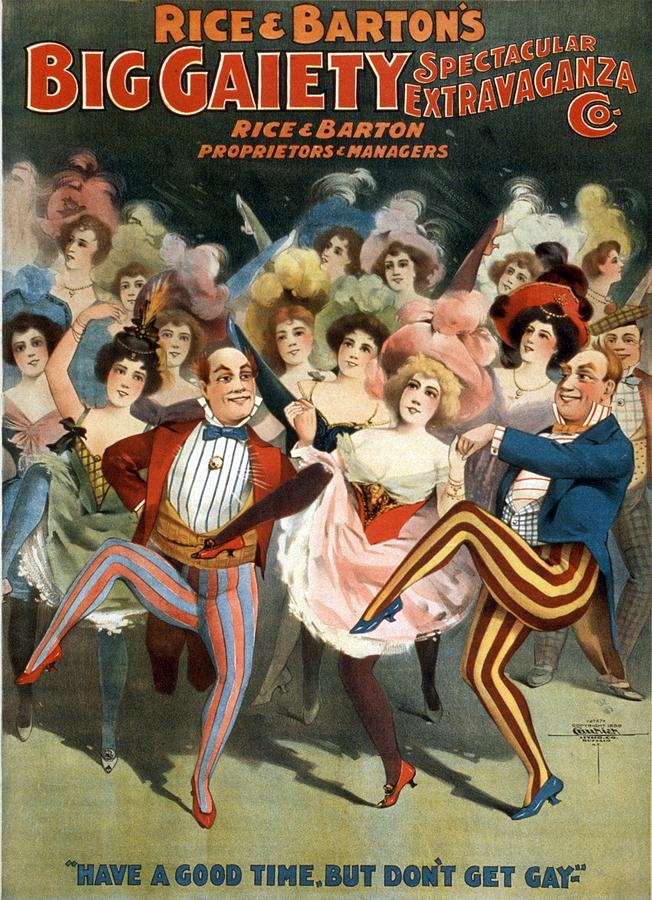This vintage poster, likely from the turn of the 20th century, promotes Rice and Barton's Big Gaiety Spectacular Extravaganza. The prominent text in bold red letters at the top reads "Rice and Barton's Big Gaiety Spectacular Extravaganza" with the words "Proprietors and Managers" underneath. The scene depicts lively dancing men and women attired in vibrant costumes. Notably, on the far right, a man is wearing yellow and red striped tights paired with high heels. Another man nearby dons blue and red striped leggings with red high heels, performing a high kick reminiscent of the can-can dance.

In the center, a bald man with red hair on the sides sports a red topcoat and vertically striped white shirt with a blue bow tie and a cummerbund. His gray and red striped tights and red ballet slippers match his energetic dance pose, leg high in the air. Beside him, a woman in a fluffy pink tutu adds to the dynamic display. The background features women in colorful dresses and flowery bonnets, possibly ballet dancers, mirroring the joyous, whimsical atmosphere.

At the bottom of the poster, on a pale green background with darker green text, a curious phrase reads: "Have a good time, but don't get gay." This whimsical and illustrative poster, with a small, unreadable artist's signature on the lower right, encapsulates the flair and excitement of the era's vaudeville shows.